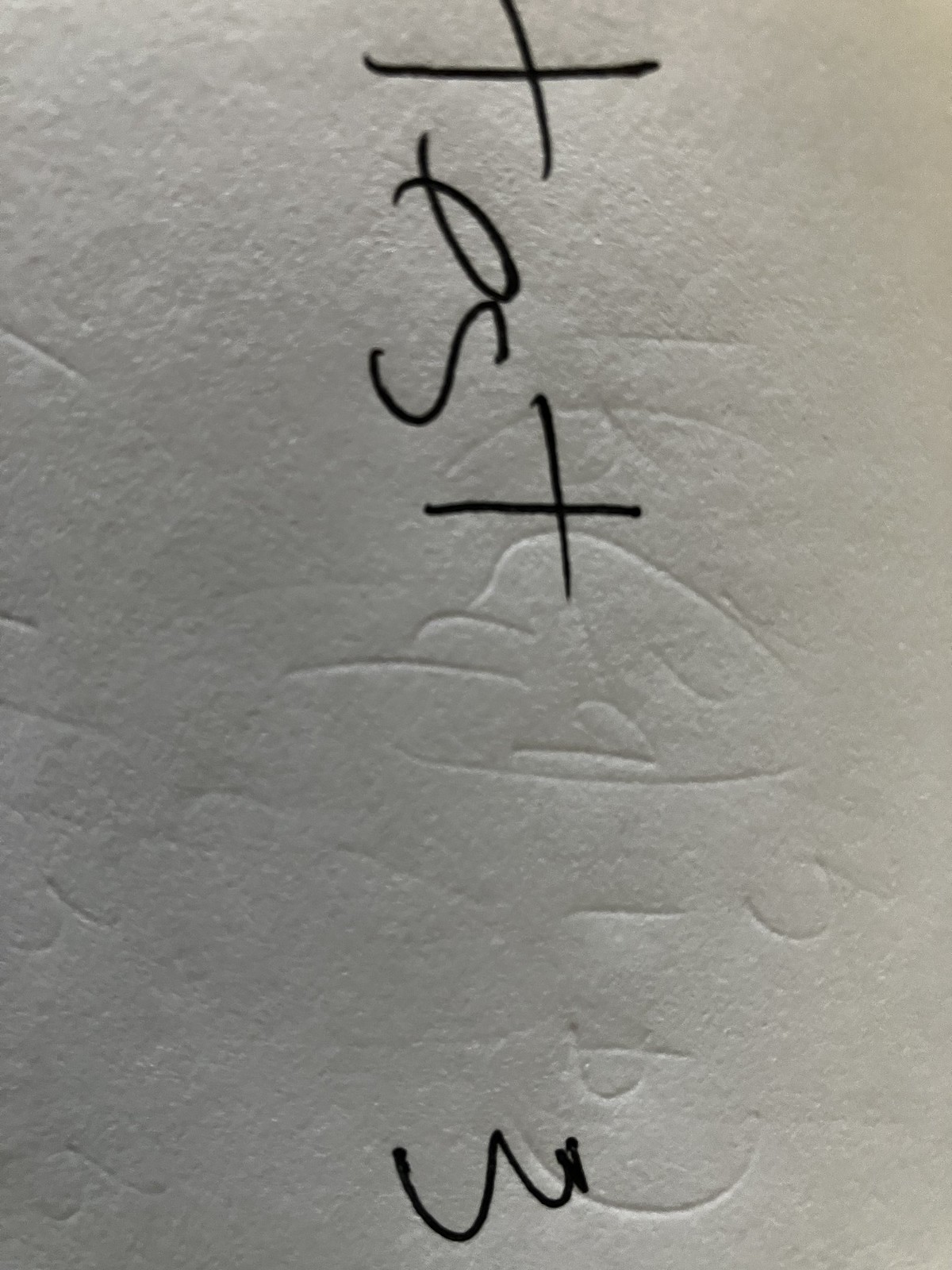This close-up photograph captures a white piece of paper with the bold, black text "TEST3" prominently displayed in the center. The paper is textured with faint impressions of various characters, including numbers like 1, 2, 3, and 4, as well as the letter B and parentheses. These impressions add depth and detail to the image, giving it a tactile quality. The arrangement of the characters around the paper appears random, suggesting a series of tests or annotations. The stark contrast between the black text and the white background draws immediate attention to the word "TEST3," making it the focal point of the photograph.